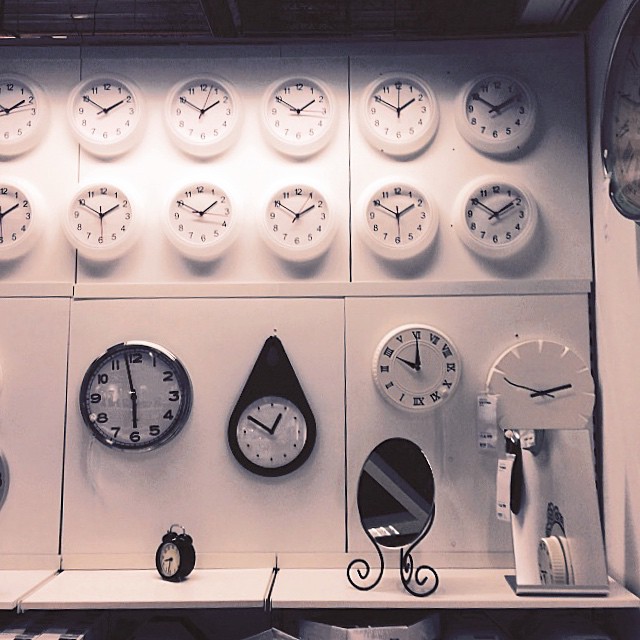This black and white photograph showcases a wall adorned with an eclectic array of clocks. Dominating the top section are 12 identical clocks neatly arranged in two rows of six, each housed in a white circular frame and all set to approximately 1:50. Below these uniform timepieces, a white shelf displays a diverse collection of clocks: 

1. A traditional alarm clock with a Mickey Mouse-styled design in black.
2. A sleek silver analog clock displaying the time as 5:58.
3. A unique clock embedded in a black teardrop-shaped frame, showing 12:50.
4. A white clock featuring Roman numerals.
5. A whimsical clock designed to resemble a basketball backboard.
6. An ornate silver mirror clock standing on a curly base.

The photograph's monochromatic palette highlights the varied designs and forms of the clocks, creating a striking visual composition.